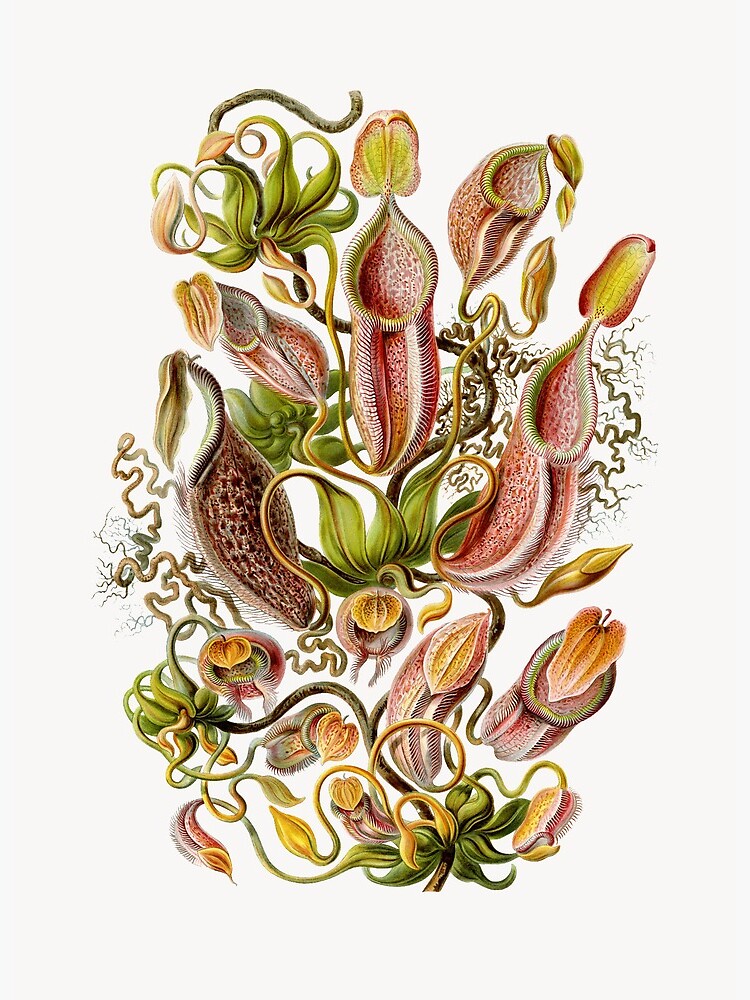This is a hand-drawn and colored painting of various carnivorous plants set against an off-white background with a gray tinge. The image depicts a central stalk from which multiple tubes and elongated cylindrical structures extend, prominently featuring plants that resemble both pitcher plants and Venus flytraps. The pitcher plants, scattered across the upper half of the drawing, have a leopard print design with brown spots on a tan lining, and their openings are capped with green lids edged in yellow. Below, smaller plants, including Venus flytraps with their distinctive green and red snapping jaws, intertwine around the main stem. The Venus flytraps are mostly closed, appearing like book pages ready to trap prey. The entire composition, roughly five to six inches high and four inches wide, showcases an intricate network of vines and tendrils, emanating from a leafy base and wrapping around the various carnivorous traps, encapsulating the fascinating nature of these insect-eating species.